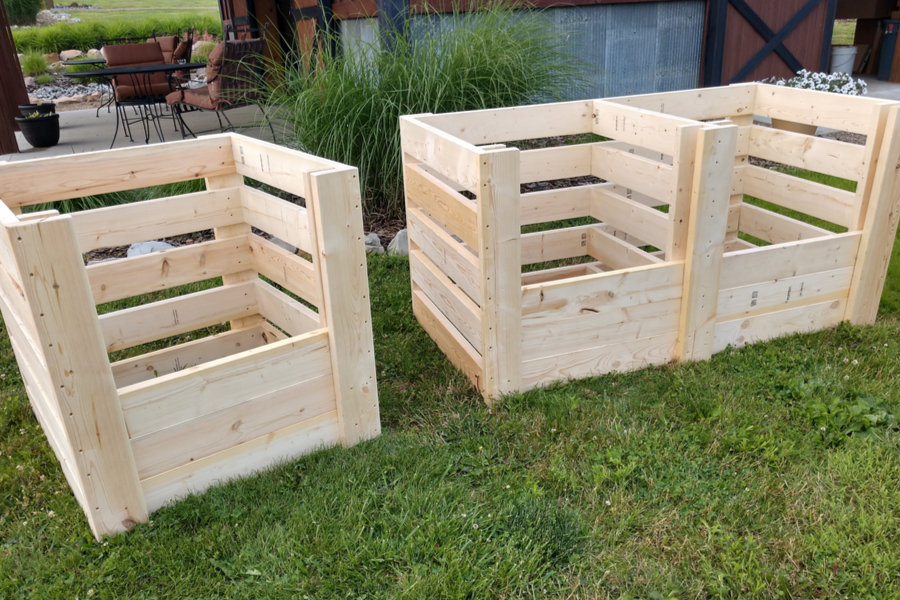The photograph captures a close-up of three square wooden crates positioned on a grassy lawn during the daytime. These crates, resembling open cages with horizontal wooden panels, are made from light pale-colored wood. On the left, a single crate stands alone, while to the right, two crates appear connected but are divided in the middle, all of similar size. Behind the crates, there's a brush of grass leading up to a patio area featuring brown wrought iron chairs with matching brown cushions and a wrought iron table. The background reveals more distinctive features, including a red structure that could be a barn or a house, characterized by a wooden door adorned with an 'X' pattern.